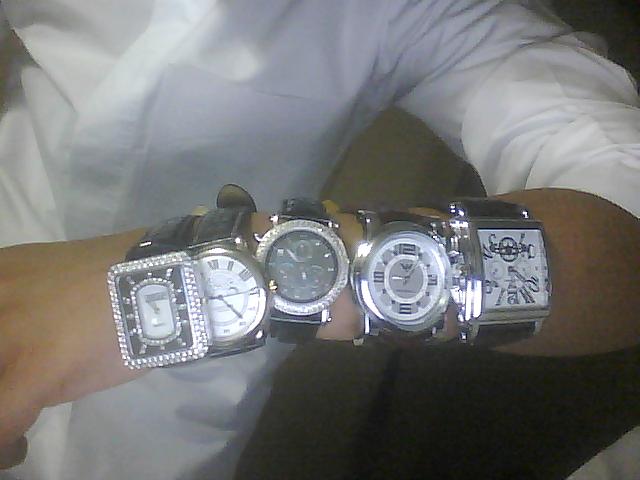This photograph captures a close-up of a man's outstretched arm, prominently displaying five different wristwatches. Dressed in a white shirt with sleeves rolled up, the man's light brown, Caucasian-toned skin contrasts against the backdrop of black, grey, and brown shades. The focus is squarely on the assortment of watches, each uniquely designed and exuding luxury. The first watch on the left features a rhinestone-studded decoration; the second resembles an antique clock face with Roman numerals. The third watch is notable for its multiple dials, while the fourth features a stylized design with the numbers 3, 6, 9, and 12 prominently displayed. The final watch presents an avant-garde aesthetic, with a seemingly chaotic arrangement of numbers. All the watches have a mix of silver and black elements, with three being circular and two square-shaped. Despite the image's slightly blurry and older appearance, the opulence and individuality of each timepiece are strikingly evident.